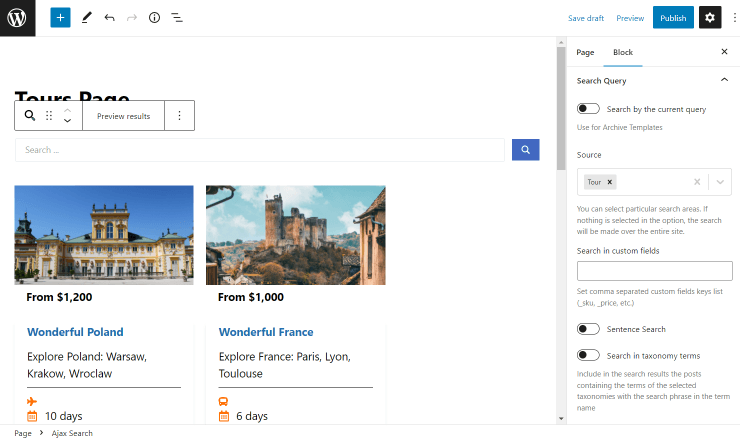The image is a horizontal screenshot of a travel website's interface. Dominating the upper left corner is a black square featuring a "W" logo and a circle. Adjacent to this is a plus button, and along the upper-right corner are icons linking to saved drafts, a preview, a publish button, and a settings button.

The screenshot is divided into two main sections. The larger, left section is set against a white background and highlights two travel deals. The left photograph, titled "Wonderful Poland," advertises trips starting at $1,200. Beside it, another photograph promotes "Wonderful France," with prices beginning at $1,000. Above these images is a horizontal text box marked "Tours Pago," complete with a search icon and a preview results button.

On the right-hand side, a narrower vertical section features a scrollbar and is split into two tabs: Page and Block. Options within this section include search query fields, source specifications, and the ability to select specific search areas, or perform a comprehensive site-wide search if no specific areas are chosen. Additionally, there is a text box for searching within custom fields. Beneath this, two small slider buttons are labeled "Sentence Search" and "Search in Taxonomy Terms." The website's background and banner maintain a clean, white aesthetic.